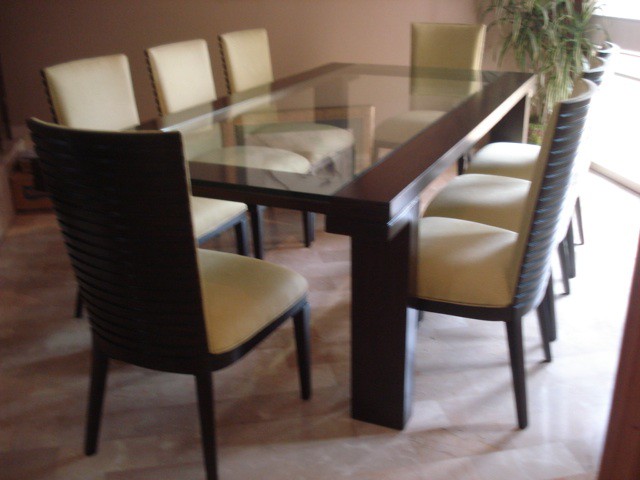This is a detailed color photograph of a modern, high-end dining set situated in a sleek indoor setting. The main feature is a large rectangular dining table with a dark mahogany wood frame that boasts clean, simple lines and a substantial, blocky structure. The tabletop is composed of a transparent plate glass, revealing reflections and offering a sleek, sophisticated appearance. Surrounding the table are eight chairs—three on each of the longer sides and one at each end. The chairs, which have dark mahogany frames like the table, are upholstered in cream-colored cushioning, extending from the seats up to the backs. The backs of the chairs feature a slightly open, carved design, which provides a contrast to the table’s bulkier profile with their thinner, lighter overall structure.

The room itself has a sandy beige or pale pink backdrop, contributing to a warm ambiance. In the upper right corner of the image, there is a lush green plant, bringing a touch of nature to the modern aesthetic. Below the table, an off-white rug with a rose pattern further accentuates the elegant setting. There is a hint of natural light streaming in from a window or glass door on the right, casting light and shadow play across the scene. The flooring appears to be a light grayish marble or stone tile, adding to the luxurious feel of the space. Overall, the photograph captures an inviting, well-designed dining area that blends modern style with comfort.